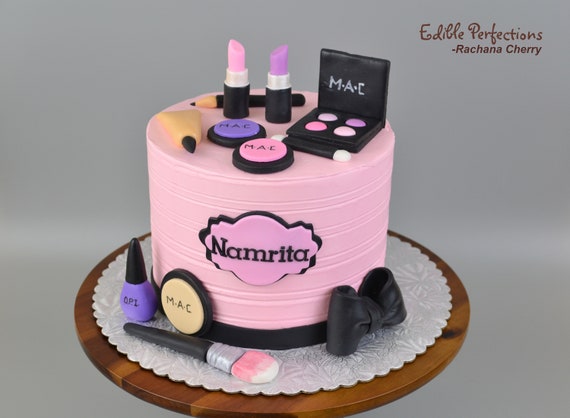This photograph captures an exquisitely designed cake, aptly titled "Edible Perfections" by Raschina Cherry. The cake, showcasing meticulous artistry, is set on a rustic wooden round surface. At the base, a delicate white lace doily adds a touch of elegance. Arranged atop the doily are a few makeup-themed decorations: a chic makeup brush in black, pink, and silver, a sophisticated black bow, a stylish black and tan MAC makeup compact, and a vibrant bottle of OPI nail polish in a rich purple shade with a black cap.

The cake itself, adorned with pink and black fondant, features the name "Namrita" elegantly inscribed in black font at its center. The top of the cake displays an impressive array of edible makeup items, including a purple and pink compact with intricate black designs, a tan tube of foundation, a pink and purple lipstick, a sleek black eye pencil, and an intricately detailed eyeshadow compact. The eyeshadow compact showcases an array of colors: light pink, purple, white, and a deeper pink, accompanied by an applicator. This cake masterfully blends culinary artistry with makeup-themed aesthetics, creating a visually stunning and delectable centerpiece.